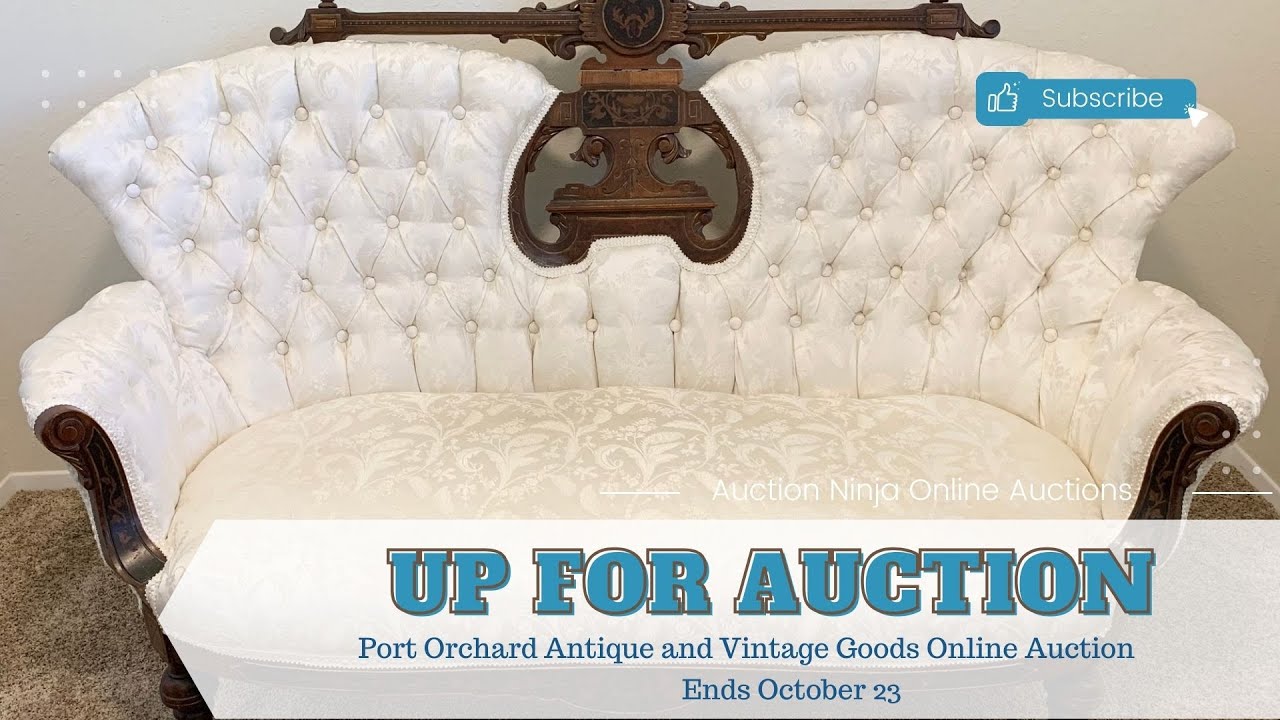This horizontal, rectangular image displays a vintage-style loveseat upholstered in shiny, white silk-like fabric with a subtle floral pattern. The backrest features a curved design with button tufting and large, round, carved wooden posts at the top, intricately detailed with a curvy, plant-like motif. The loveseat has armrests that extend outward, and a distinctive wooden inlay divides the two seats. The piece is situated in a room with white walls and carpet. In the lower right corner of the image, a white box with bold blue lettering announces, "Up for Auction," followed by smaller blue text stating, "Port Orchard Antique and Vintage Goods Online Auction," with the auction ending on October 23rd. This suggests that the loveseat is available for online bidding.